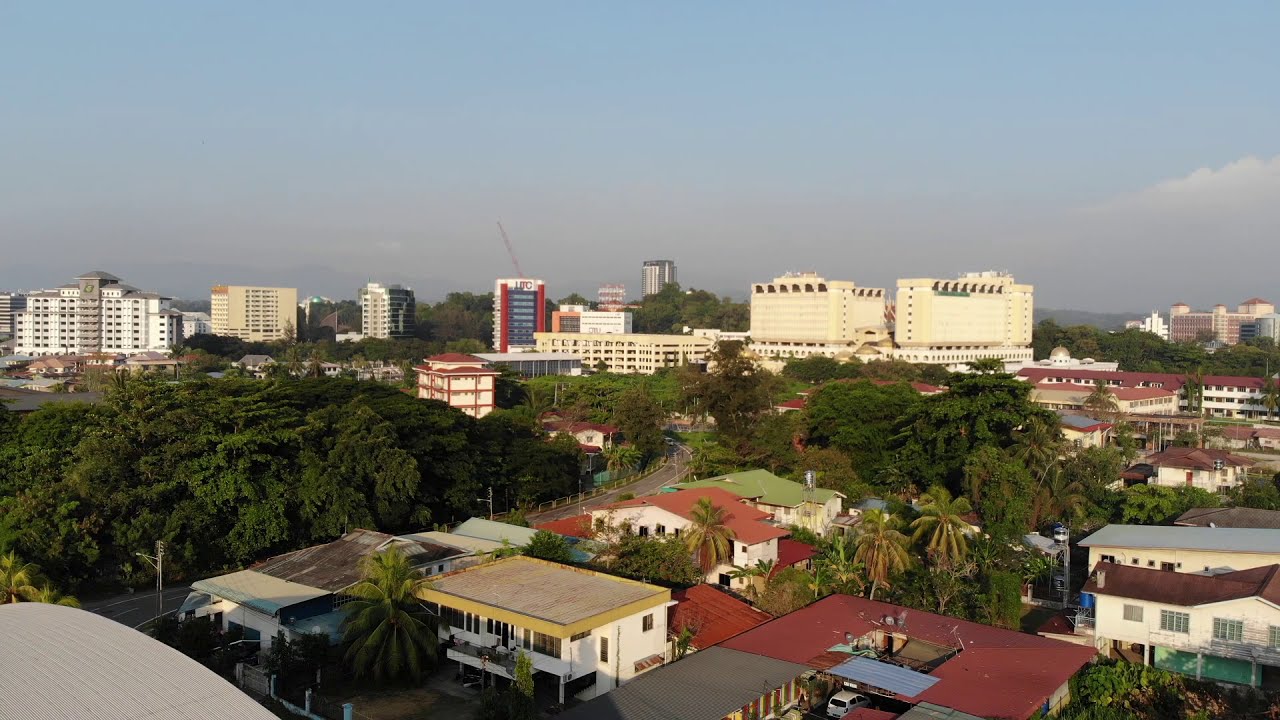The photograph captures a vibrant cityscape, seemingly in a tropical locale, suggested by the numerous palm trees scattered throughout the scene. Dominating the background are high-rise buildings, particularly on the center-right where two tall, white rectangular structures stand prominently. Adjacent to these on the left, there's a multi-story parking garage followed by a red building with blue windows. Further left, another high-rise, resembling a motel with many windows, completes the skyline. A crane looms in the distance, hinting at ongoing development.

In the foreground, a cluster of low-rise buildings, likely residential homes, display varied colored roofs—red, blue, green, and white—adding a splash of color to the otherwise muted palette of the skyscrapers. A road weaves through this residential area from the left edge of the image to the right, bordered by dark green trees that enhance the lush environment. The bright pale blue sky, adorned with thin, hazy clouds, indicates a sunny day. This detailed view is taken from an elevated vantage point, providing a comprehensive look at both the bustling business district and the serene residential neighborhood.